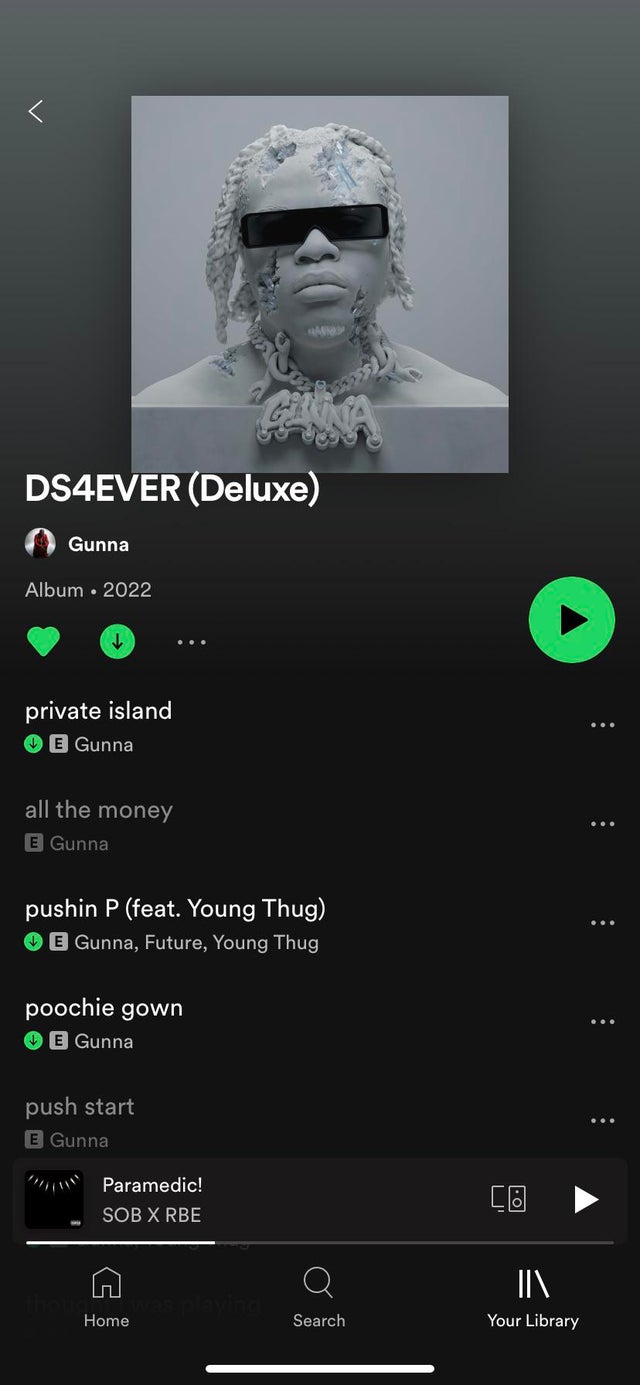A detailed screenshot of a mobile device displaying a playlist with a predominantly black background. The featured album is "DS Forever Deluxe," released in 2022. The album cover showcases a serious-looking African-American man wearing sunglasses and a large gold necklace. The list of songs visible on the screen includes "Private Island," "All the Money," "Pushin' P," and "Push Start." At the bottom of the screen, navigation icons for Home, Search, and Library are clearly displayed.